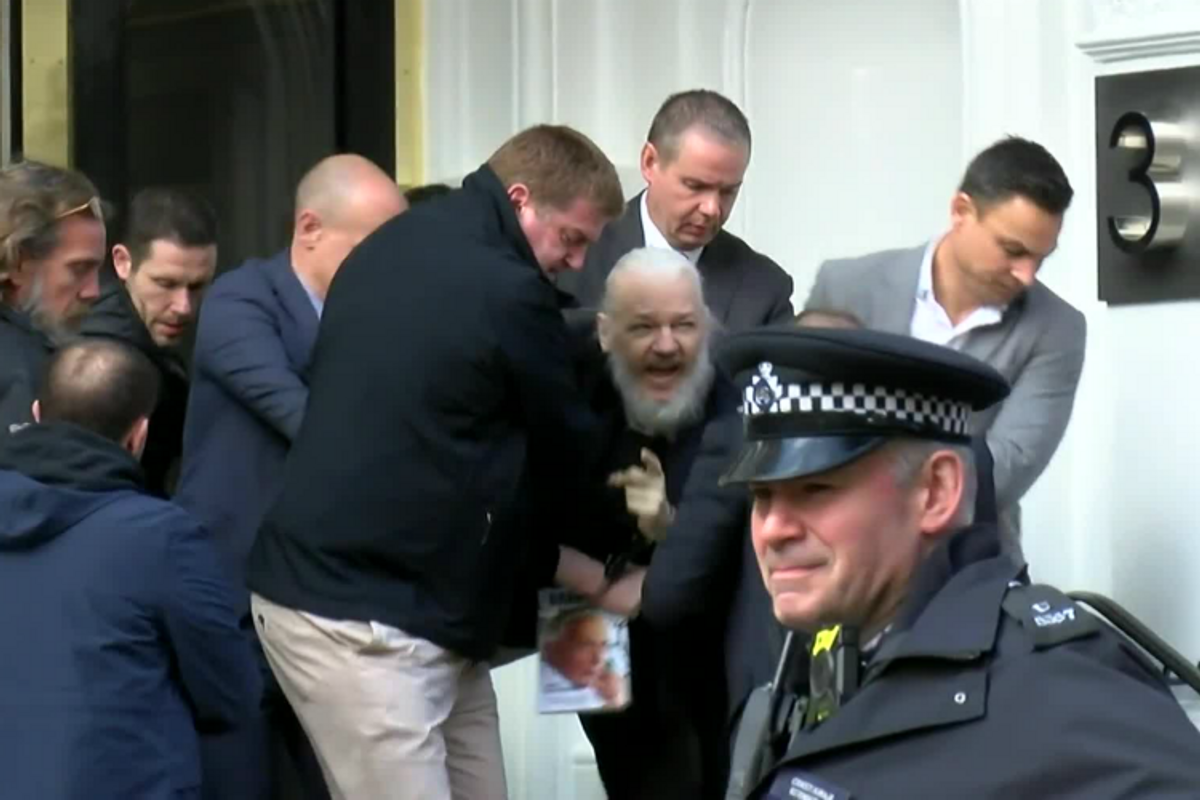The photograph captures a dramatic moment involving Julian Assange, who appears to be in the process of being arrested. Assange, with a pale yellowish complexion and a long white beard, stands at the center of the image. His mouth is open as if he is shouting or protesting, and his left hand points outward, suggesting defiance or resistance. Surrounding him are several men in suits and dark jackets; two of them are notably strong and middle-aged, restraining Assange to prevent him from moving. One of them is holding on to him more firmly, indicating the seriousness of the situation. Assange’s wrists are bound with handcuffs, visible in the photograph, reinforcing the notion of his arrest.

In the foreground, a British police officer, distinguishable by his cap adorned with a black-and-white checkered strap, stands out. He wears a gray uniform with epaulets and appears to be looking off to the side, possibly assessing the situation or observing other activity. The scene is set against a backdrop where the number "3" is visible, likely an address on a wall, providing a contextual detail. The overall composition of the photograph suggests tension and urgency, capturing a pivotal and contentious moment.